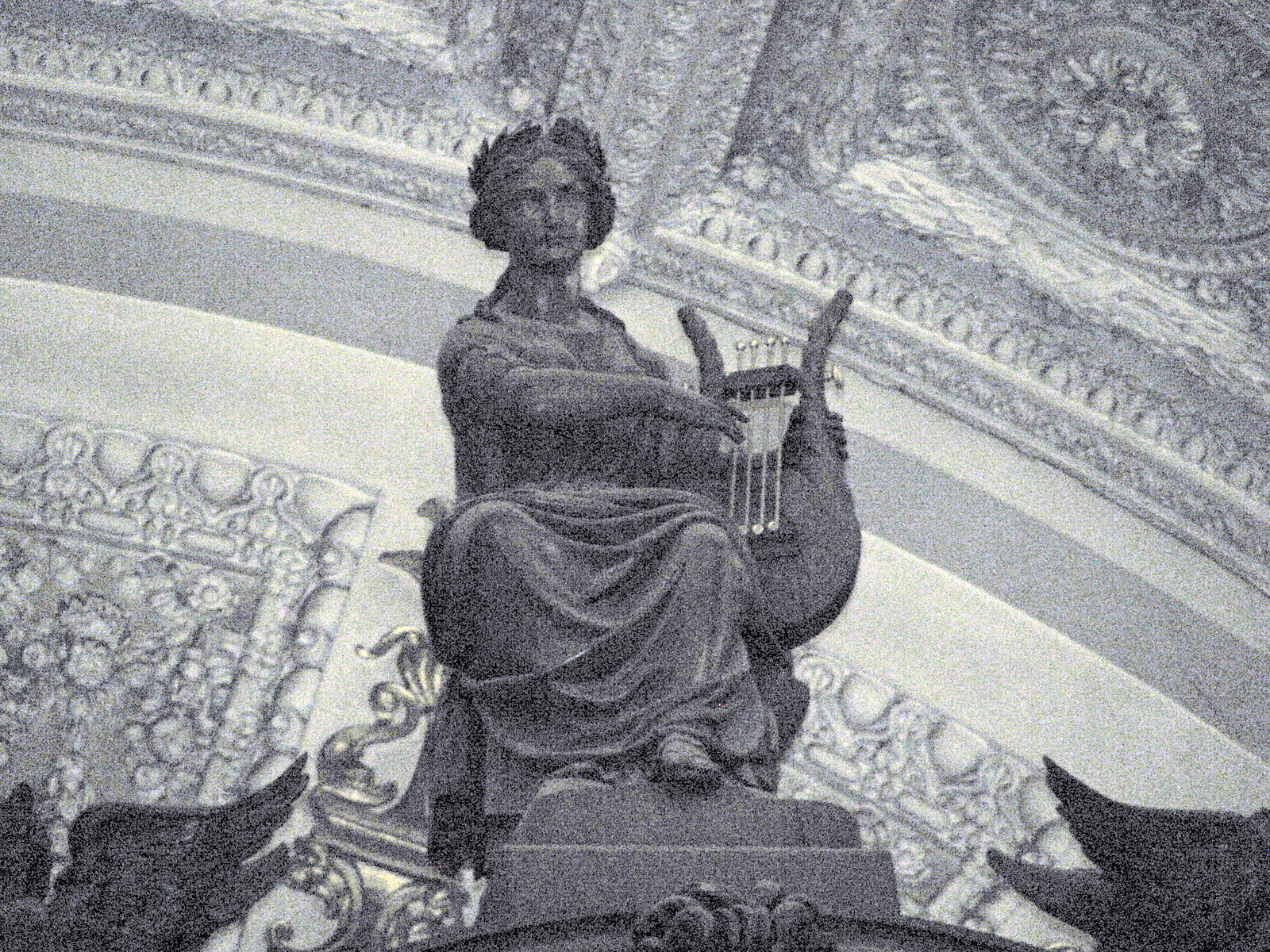This intricate and slightly blurry black and white image features a historic and statuesque scene, seemingly set within a grand cathedral or historic Italian building. Dominating the middle of the photo is a detailed statue of a woman, who might be an angel, adorned with a wreath around her head and garbed in a long, flowing dress. She is seated, holding a small four-stringed harp in her left hand, with her right hand poised to strum it. Adding to her celestial appearance, she has angelic wings visible on either side. The background reveals an elaborate, hand-carved ceiling or wall rich with historic and artistic elements, including various carvings that resemble chalices and other intricate designs. The ceiling appears white and gray, providing a stark, detailed canvas that further enhances the statue's prominence. The blend of these elements creates a striking portrayal of classical art and architectural grandeur.